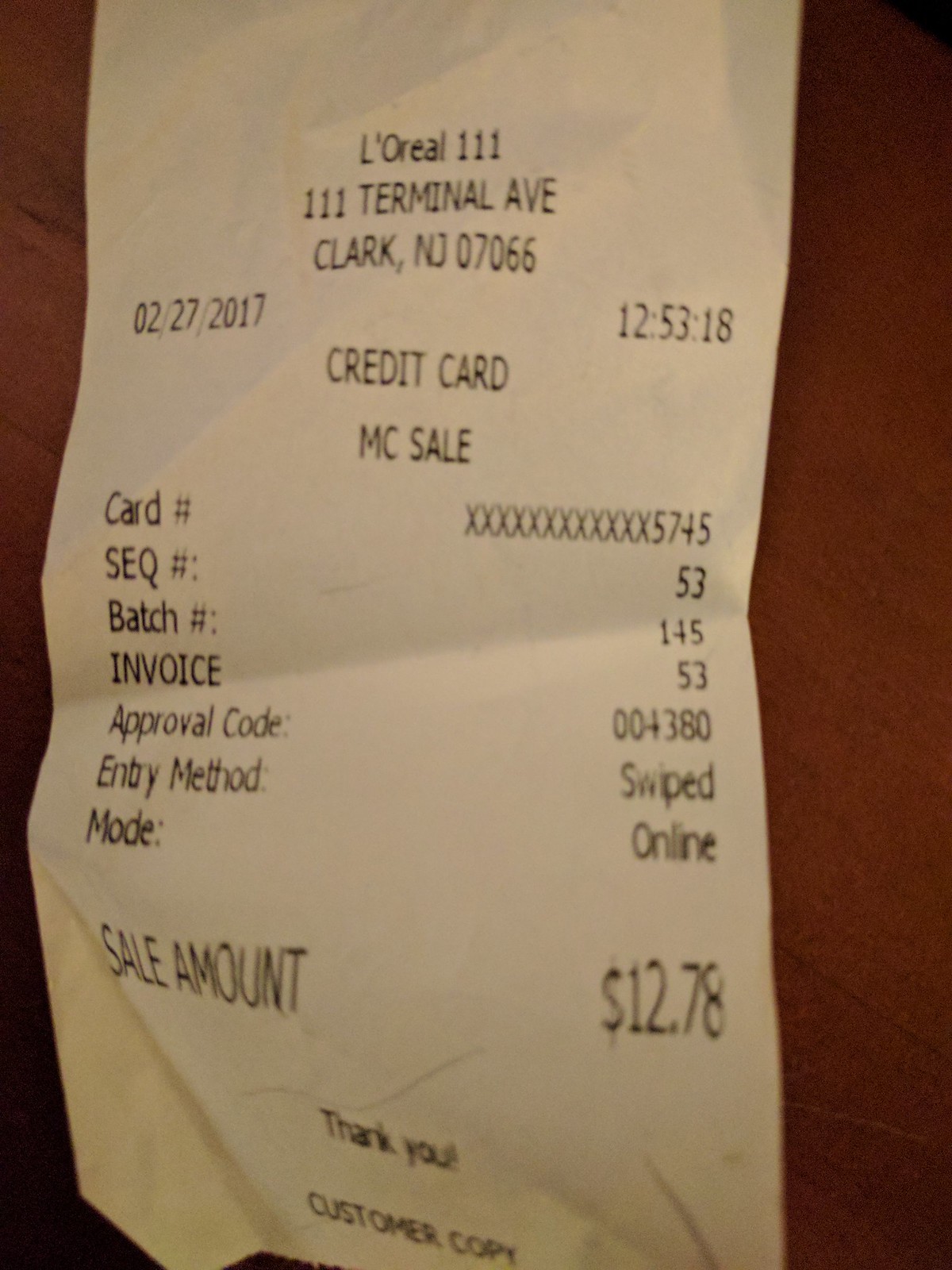This image features a close-up photograph of a long, skinny, white receipt, somewhat crumpled but still legible, placed on a brown table surface. The receipt documents a credit card sale conducted at L'Oreal, located at 111 Terminal Avenue, Clark, New Jersey, 07066. The transaction took place on February 27, 2017, at exactly 12:53 and 18 seconds p.m. The sale, made with a MasterCard ending in 5745, bears batch number 145 and invoice number 53, with an approval code of 004380. The purchase was processed by swiping the card in online mode for a total amount of $12.78. At the very bottom of the receipt, it reads "Thank you" followed by "Customer copy."